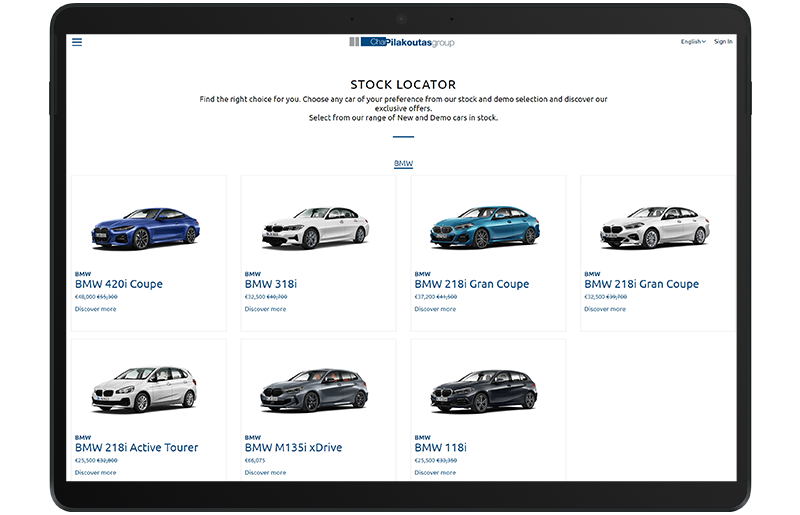Screenshot of a mobile stock locator app displaying multiple BMW car models. The user interface is framed in black and starts with language selection ("English") followed by a "Sign In" option. Below, a header reads "Stock Locator: Find the right choice for you," inviting users to choose from a stock and demo selection of cars and discover exclusive offers.

Displayed are various BMW models with the option to "Discover more" beneath each:

1. **BMW 420i Coupe** - Featured in a striking blue color.
2. **BMW 318i** - Presented in a classic white hue.
3. **BMW 218i Grand Coupe** - Also in white.
4. **BMW 218i Grand Coupe** - This variant is in teal.
5. **BMW 218i Active Tour** - An SUV version, showcased in white.
6. **BMW M135i All-Wheel Drive** - Displayed in a shipyard gray color.
7. **BMW 118i** - Appearing in a sleek black finish.

The last three models, including the 218i Active Tour and the M135i All-Wheel Drive, fall into the SUV category.